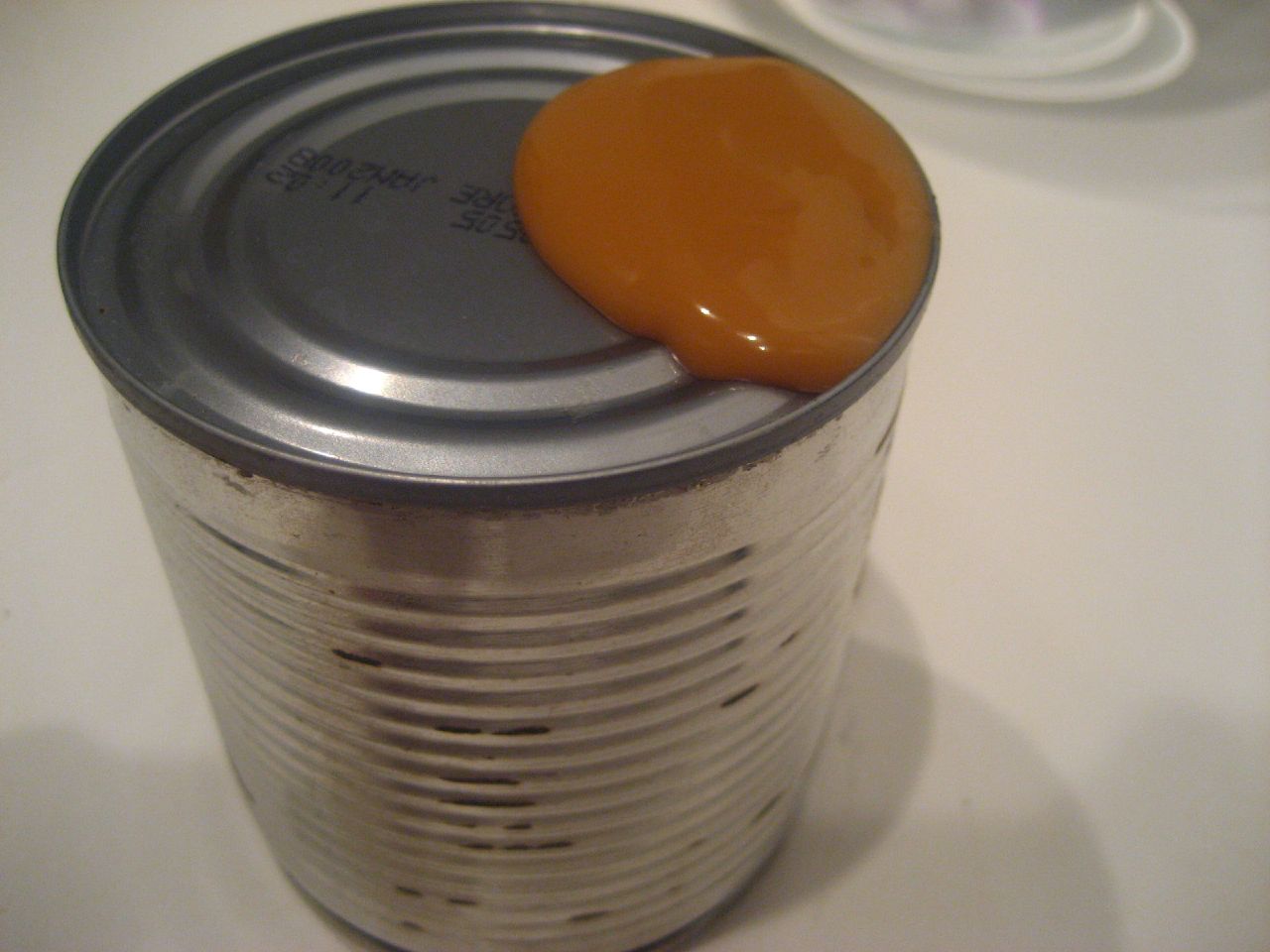This photograph captures an unlabeled aluminum can standing upright on a white countertop. The can, displaying distinct silver ridges around its circumference, has no label, revealing its metallic texture entirely. At the top of the can, there are silver rings and black text stamped with dates and numbers, including an upside-down expiration date that reads "11-02-Jan-2008." On the right side of the lid, there is a glob of caramel-colored substance, likely sweetened condensed milk that has darkened to a caramel hue, suggesting possible puncturing and oozing. The surface around the can is unevenly lit, with soft shadows indicating varied lighting, and a faint reflective object in the background hints at additional elements in the scene. There are also some rusty spots on the can, adding to its detailed appearance.